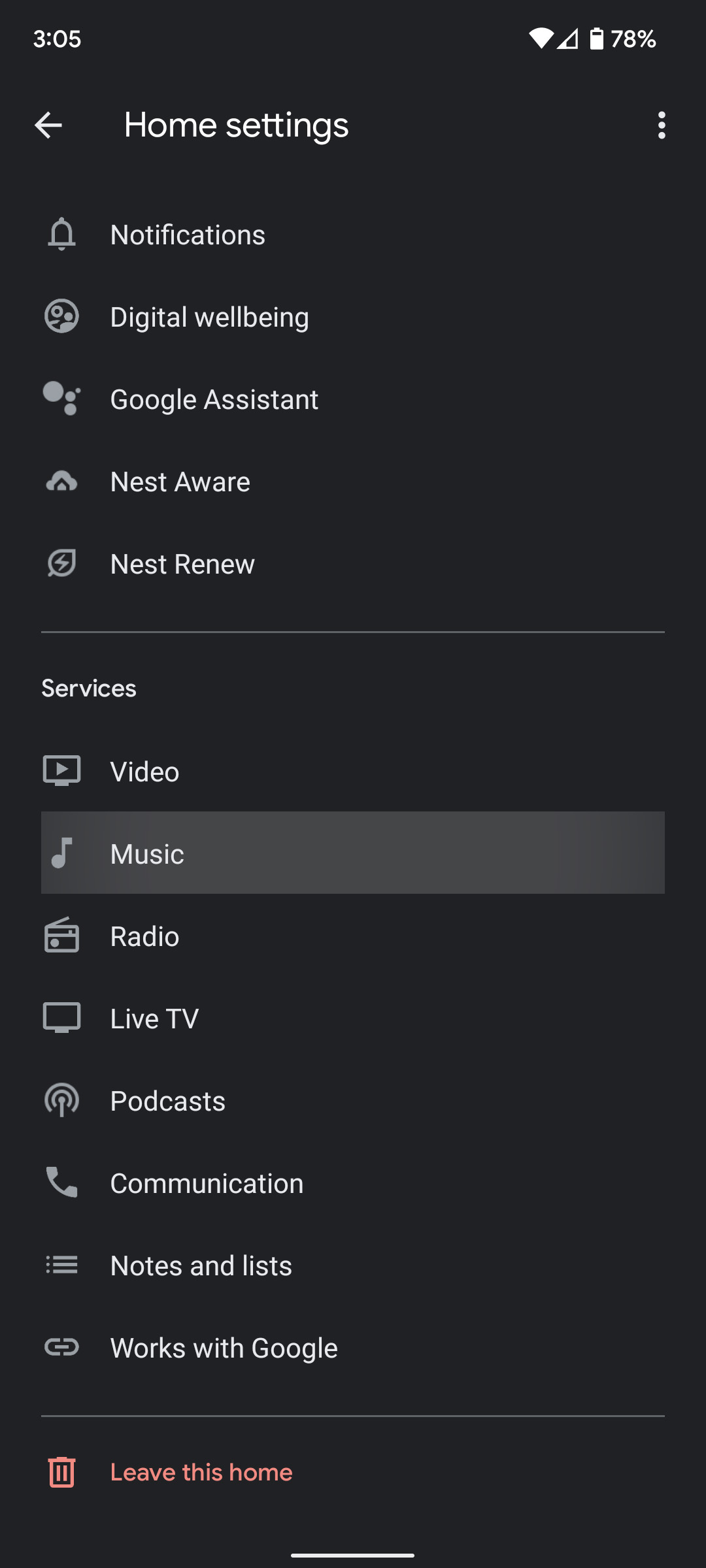The screenshot depicts a smartphone display featuring a black background accented with white text and various grey elements. At the very top of the screen, typical cell phone indicators are visible. In the upper left corner, the time reads "3:05," while the upper right corner displays wireless connectivity icons alongside a battery icon showing a 78% charge.

Directly below these indicators, a title bar labeled "Home Settings" appears, flanked by a back arrow on the left, which allows navigation to the previous screen. On the far right of this title bar, three vertical dots offer access to additional settings or options.

Subsequent to the title bar, the screen is divided into two main sections, each separated by thin grey lines. The first section is labeled "Home Settings" and lists five clickable options: Notifications, Digital Well-being, Google Assistant, Nest Aware, and Nest Renew, each paired with relevant icons.

Following the first thin grey divider, the second section is titled "Services" and contains eight options, each indicated by corresponding icons. This list begins with Video and continues with Music (currently highlighted in dark grey), followed by Radio, Live TV, Podcasts, Communication, Notes & Lists, and Works with Google.

A second grey line separates this from the final area. Near the bottom, a line of text appears, either green or red, reading "Leave this home," accompanied by a trash can icon. The display concludes with a small white line at the very bottom.